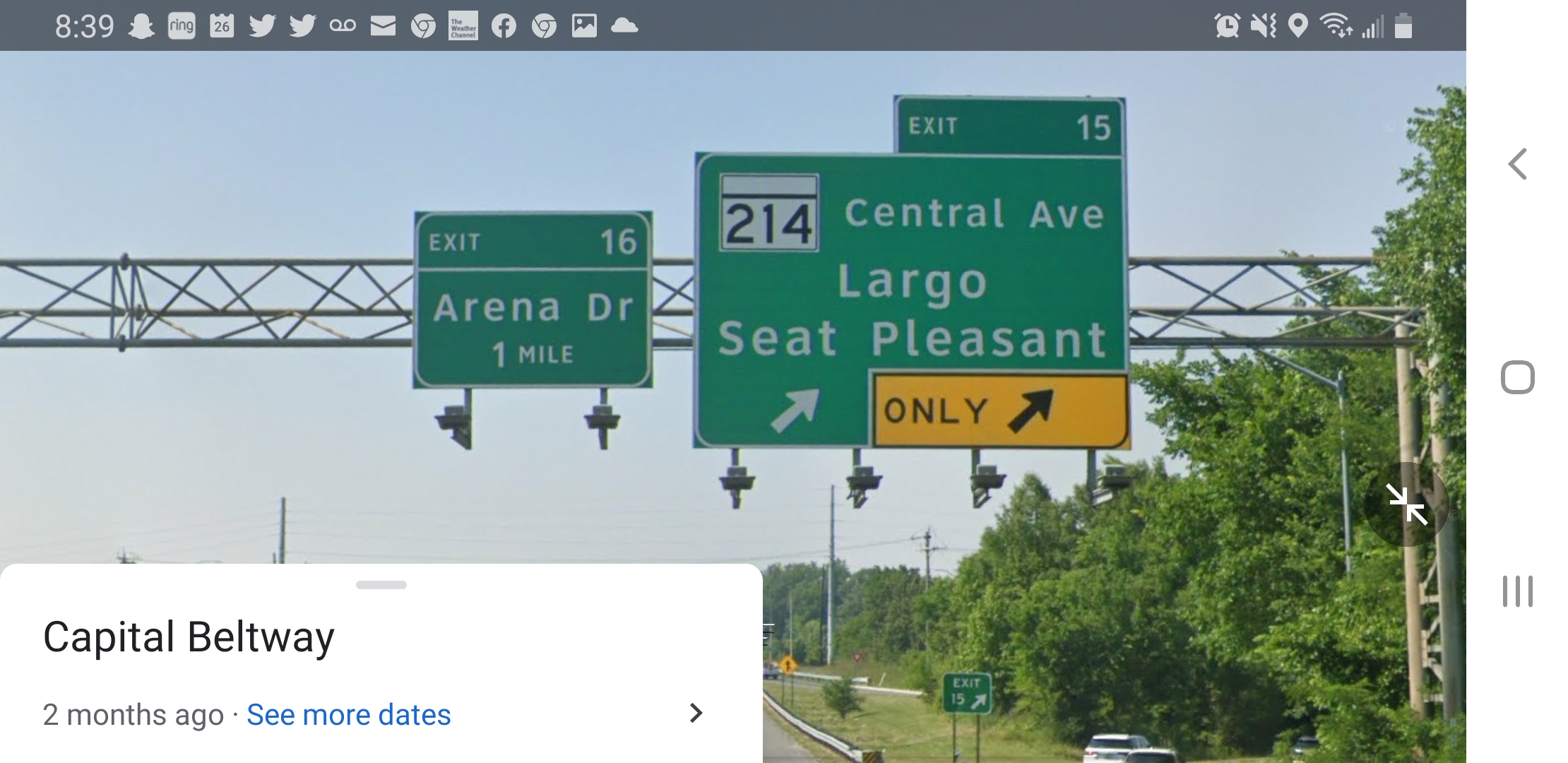This image is a screenshot, likely taken from a tablet, featuring the familiar interface icons along the top gray strip including the time (8:39), and icons for Snapchat, Twitter, email, Facebook, an alarm clock, Wi-Fi signal, and battery status. The screenshot appears to be from Google Street View, indicated by the "Capital Beltway, two months ago" label in blue on the lower left corner. 

The main focus of the image is a section of a highway with overhead green road signs. One prominent sign reads "214 Central Avenue, Largo, Seat Pleasant" in white text, and is marked as Exit 15 at the very top. It also has an oblong orange area at the bottom with the text "Only" and a right-pointing arrow. To the left of this sign, another overhead sign indicates "Exit 16, Arena Drive, one mile." The scene depicts a typical segment of the Capital Beltway with clear guidance for upcoming exits.